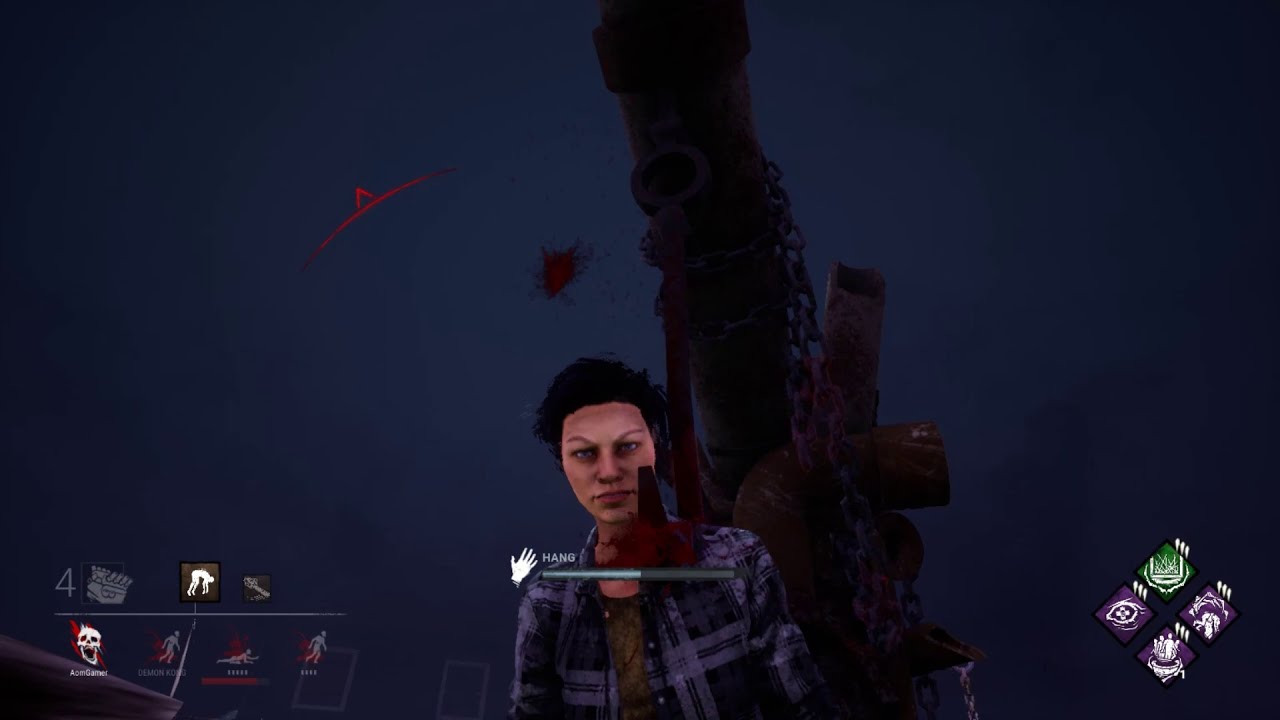In this detailed screenshot from a video game, the central focus is a character positioned toward the bottom of the screen, looking straight at the camera with a serious expression. The character, who has short black hair, is wearing a black and grey colored shirt. Behind the character, there is a large rusted metallic machine, brown in color with chains draped around it. The background of the image features a dark navy blue hue.

In the foreground, a white hand icon that reads "Hang" is prominently displayed, with a partially filled blue status bar beneath it. The bottom of the screenshot is populated with game interface elements: in the bottom-left corner, there is text that says "four" alongside several game icons, including a skull and what appears to be walking or running icons. On the bottom-right, four diamond icons are visible with varying colors — one green and three purple with white designs in the middle. Additionally, there is a red arrow indicator pointing toward the upper left near the character's head.